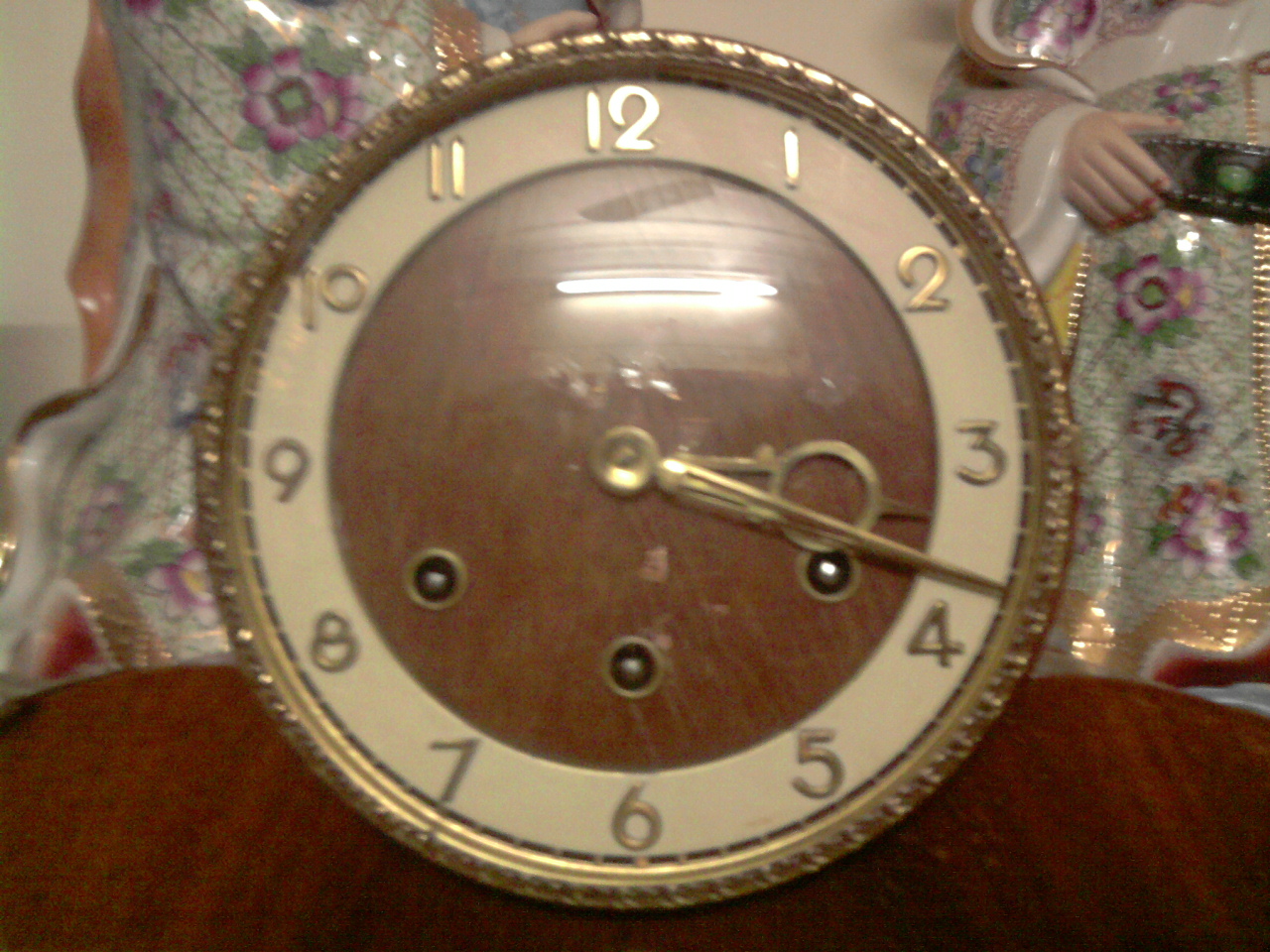A lavish close-up of a round antique clock captures its luxurious gold frame perched elegantly atop a polished wooden table. Flanking the clock on both the left and right are two exquisite ceramic figurines, adorned in traditional Chinese attire, each embellished with purple flowers entwined with lush green leaves. The clock's face is a harmonious blend of rich materials: its center boasts a wooden texture, while the surrounding area, where the finely detailed gold numbers are displayed, is an ivory hue. The golden hands of the clock, with the hour hand featuring an ornamental circle and the minute hand appearing as a sleek gold line, precisely indicate the time as 3:18. Three decorative gold circles accentuate the dial, positioned strategically—one near the four, one above the six, and another to the right of the eight. A faint reflection of a light fixture can be seen below the twelve, adding a subtle hint of modernity to this timeless piece.